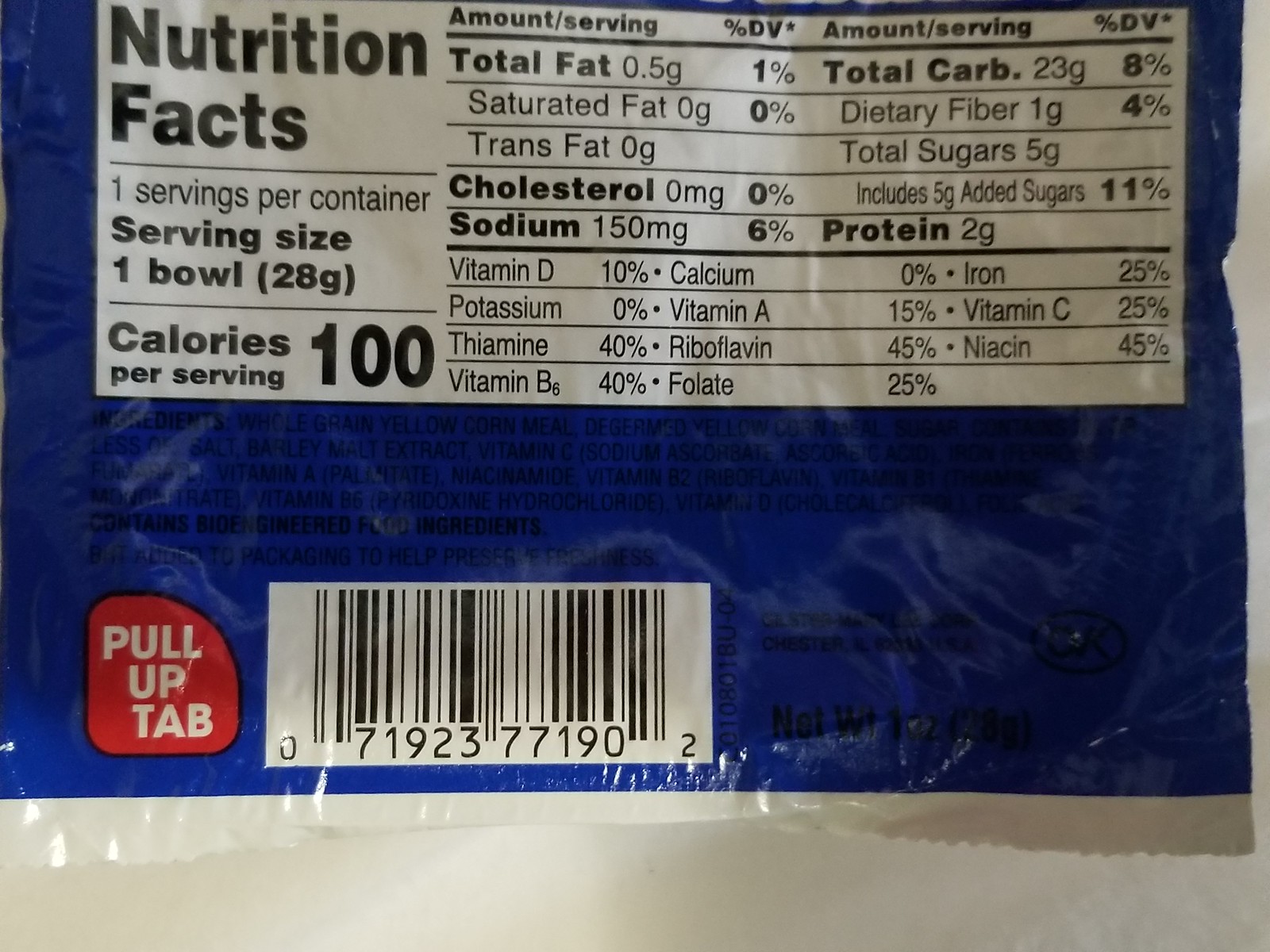This color photograph depicts the back of a flexible food packaging bag, dominated by a white nutritional facts label with black text. The label informs that a serving size is a bowl weighing 28 grams, with one serving per container. Each serving provides approximately 100 calories, with a minimal 0.5 grams of total fat, zero cholesterol, and 150 milligrams of sodium. The total carbohydrates amount to 23 grams, and there are 2 grams of protein. The label also details various vitamins and minerals.

On the bottom half of the package, essential information continues with an ingredients list and a UPC barcode. Notable ingredients include whole grain yellow cornmeal and de-germed yellow cornmeal, suggesting the product could be corn chips or a corn-based porridge like grits. A distinctive red, almost circular tab in the bottom left corner, marked with white text, instructs to "Pull-Up Tab" for easy opening. The overall packaging is primarily blue, accentuating the monochromatic black and white nutrition details and ingredients list.